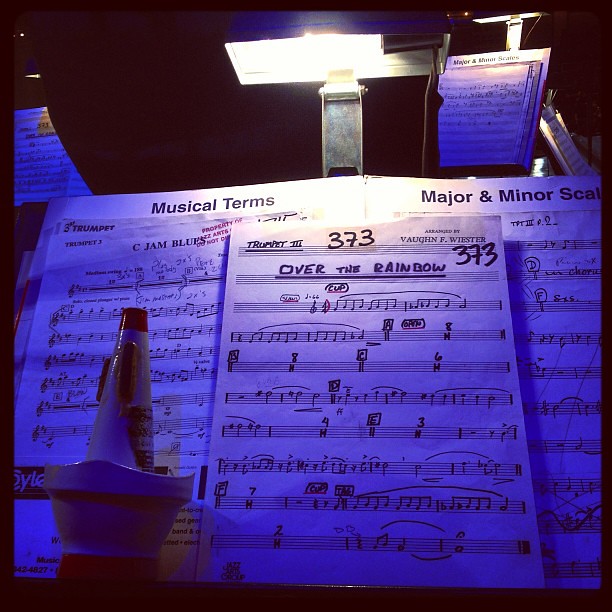The image depicts a series of music sheets illuminated by a desk lamp above them, casting a white light on the papers while a bluish-purple light fills the background, suggesting a performance or practice room. In the distant background, numerous music stands are visible, each with attached lights, indicating multiple musicians potentially preparing for a session. The music sheets in focus are spread across a stand, with the left page titled "C Jam Blues" featuring seven or eight musical lines. Superimposed over it, the middle sheet titled "Over the Rainbow" includes eight lines of music with the number "373" written above it. The right page lacks a visible title but contains about ten lines of musical notation. The background text indicates topics such as "musical terms" and "major and minor scales." The composer’s name, "Vaughn E. Weister," is noted near the bottom, suggesting these are trumpet pieces. There is a slight orange tint near the foreground, but overall the room is dimly lit with dominant hues of white and blue-purple. These sheets are actual musical notations rather than tablatures, contributing to a detailed and authentic practice setting.